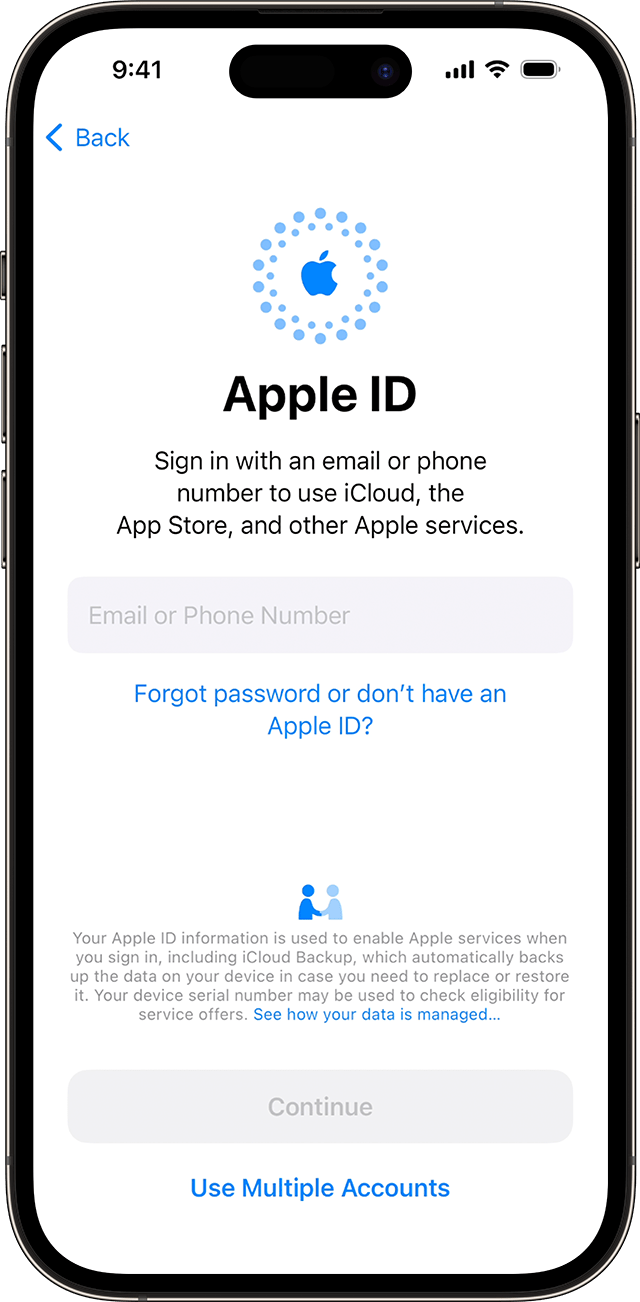This image features a detailed screenshot of an Apple iPhone's front interface, likely depicting the initial setup or sign-in screen for an Apple ID. The iPhone's sleek silver edges and the placement of the buttons on the left and right sides clearly indicate it is an Apple device. 

In the center of the phone's screen, set against a white background, is the text "Apple ID" displayed prominently in black letters. Positioned above this text is the distinguishable Apple logo. Just below "Apple ID," there is an informative message instructing users to sign in with an email or phone number to access iCloud, the App Store, and other Apple services.

Centrally located on the screen is a text box labeled "Email or phone number," inviting users to input their details. Directly underneath this box is a bright blue hyperlink reading, "Forgot password or don't have an Apple ID," providing additional support options.

Towards the lower portion of the screen is an icon depicting two people shaking hands, followed by an explanation about how the Apple ID information will be used. Beneath this, a "Continue" button is visible, though it is currently grayed out, indicating that more information is required before proceeding. 

At the very bottom of the screen, another blue hyperlink labeled "Use multiple accounts" suggests an option to manage multiple Apple ID accounts, which redirects users to a different page upon clicking. 

Finally, in the top left corner of the screen, the word "Back" in blue letters accompanied by a leftward-facing arrow provides a navigation option to return to the previous screen.